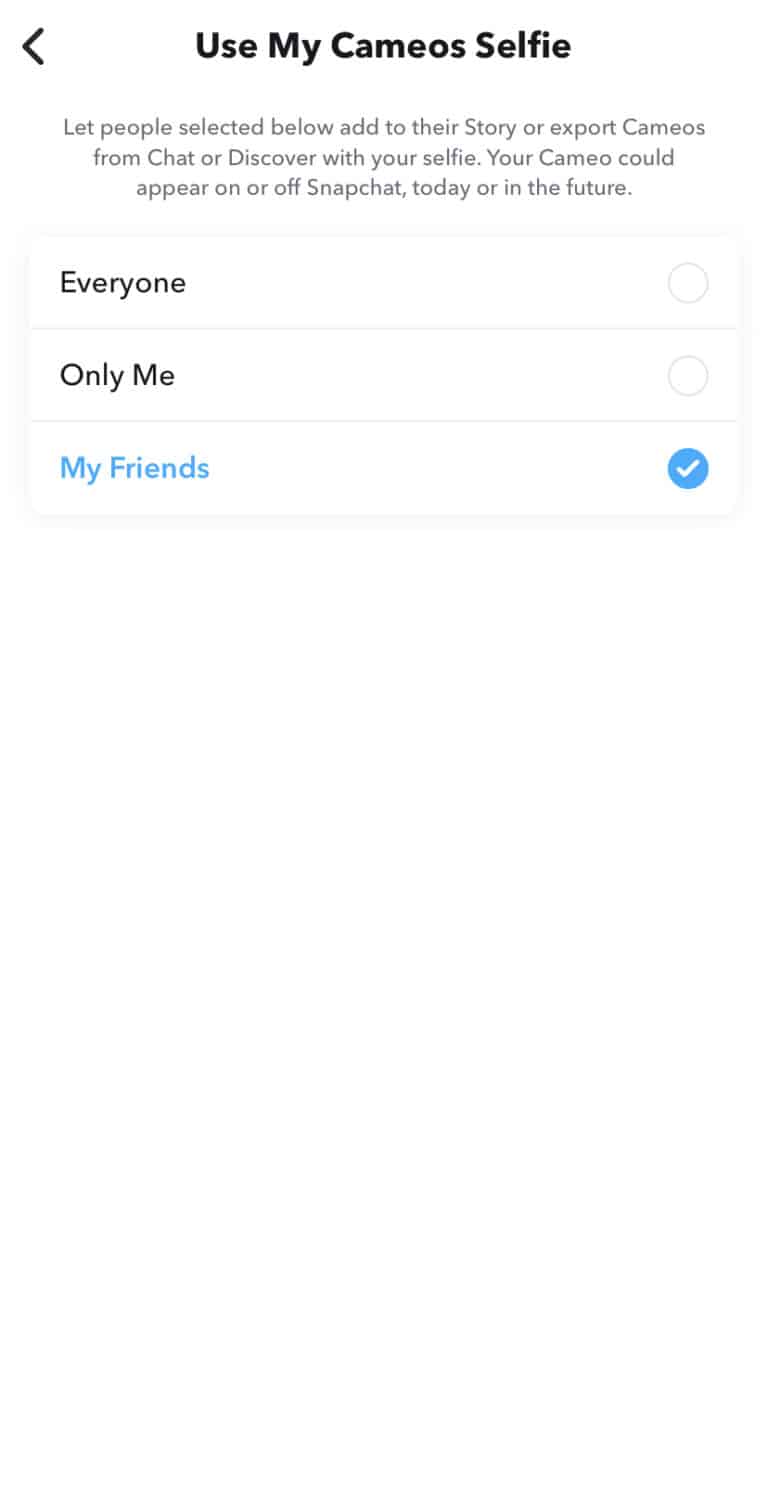In the image, prominently displayed at the top center, the phrase "Use my Cameos Selfie" is written in bold, black text. To the left of these words is a left-pointing arrow, also in a bold style. Just below this title, in smaller, light gray text, is the instruction: "Let people selected below add to their story or export Cameos from chat or Discover. With your selfie, your Cameo could appear on or off Snapchat today or in the future."

Following this, the image contains a section of selectable options presented in a boxed format. The first box reads "Everyone" on the far left in dark black text. To the far right of this box is an empty circle with a white background. The second box down reads "Only Me," again in black text, with another empty circle on the far right against a white background. The final box in this section reads "My Friends" in light blue text, and on the far right, instead of an empty circle, there is a filled blue circle containing a white checkmark, indicating that this option is selected.